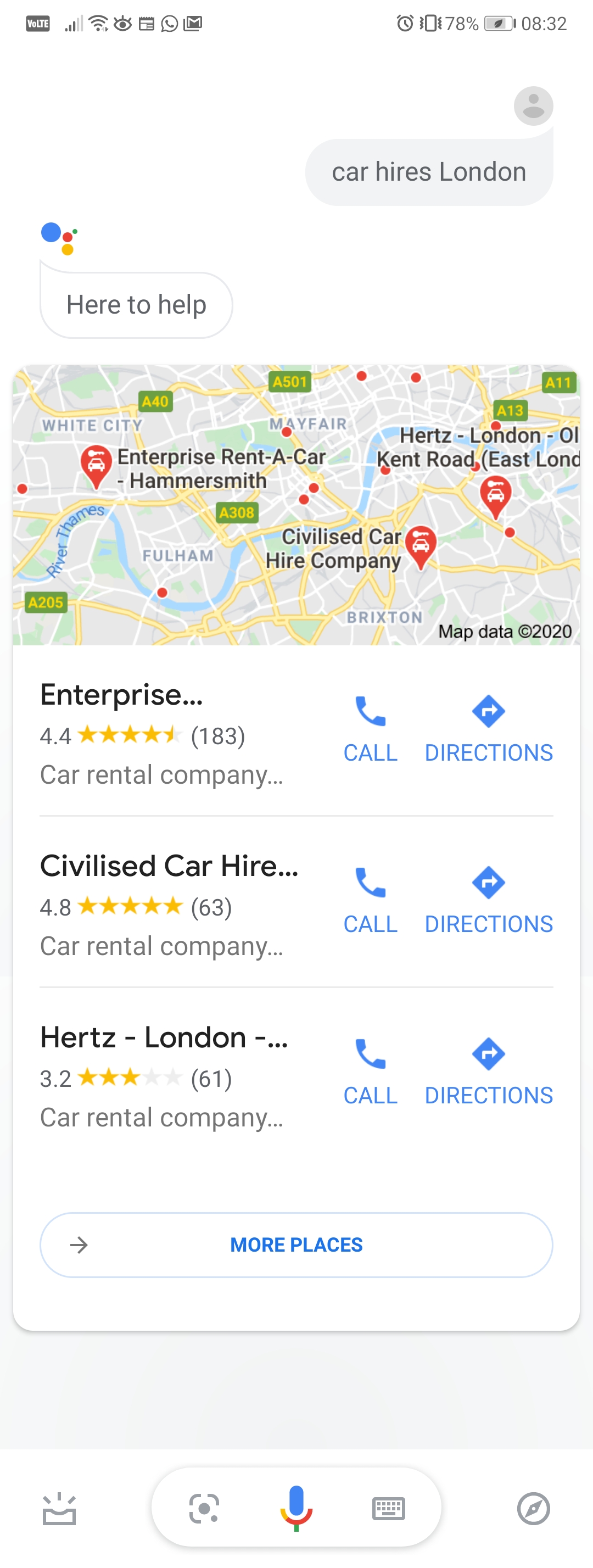**Detailed Description of the Image:**

The image is a vertically oriented rectangular layout on a white background, displaying various informational elements. At the top of the image, there are status icons typically found on a mobile device, including battery life at 78% and the time displayed as 08:32. 

Towards the right side beneath the top icons, there is a light gray rectangular oval with the text "Car hires London" in a darker gray font.

On the left side below the icons, there are a few colored dots followed by a speech bubble in gray font that reads "Here to help" on a white background.

Below this section, the image transitions into a new vertical rectangular area that features a map at the top. The map includes several lines in yellow and blue, representing routes. There are points marked with text in bold black font, including:
- "Enterprise Rent-A-Car Hammersmith"
- "Civilized Car Hire Company"
- "Hertz Kent Road"
- Another point that is partially cut off on the right side.

Under the map, three listings provide detailed information about car hire companies:
1. **Enterprise...**
   - **Rating:** 4.4 with four and a half yellow stars (183 reviews)
   - **Actions:** To the right, a turquoise phone icon with "CALL" and a diamond with a right arrow followed by "DIRECTIONS" in all caps.

2. **Civilized Car Hire...**
   - **Rating:** 4.8 with five yellow stars (63 reviews)
   - **Actions:** Similar to the first listing with "CALL" and "DIRECTIONS" in turquoise, and the additional description "Car rental company" under the stars. Note: "Civilized" is spelled with an "S."

3. **Hertz - London...**
   - **Rating:** 3.2 with three yellow stars (61 reviews)
   - **Actions:** Again features "CALL" and "DIRECTIONS" in turquoise, with "Car rental company" under the stars.

At the bottom of this vertical area, a white horizontal oval contains a small gray arrow pointing to the right on the left edge, and "MORE PLACES" in the center in all caps and turquoise font.

Further down, the image has an off-white area followed by more icons at the very bottom. Central among these is a microphone icon with a turquoise speaking part, accompanied by other multi-colored elements beneath it.